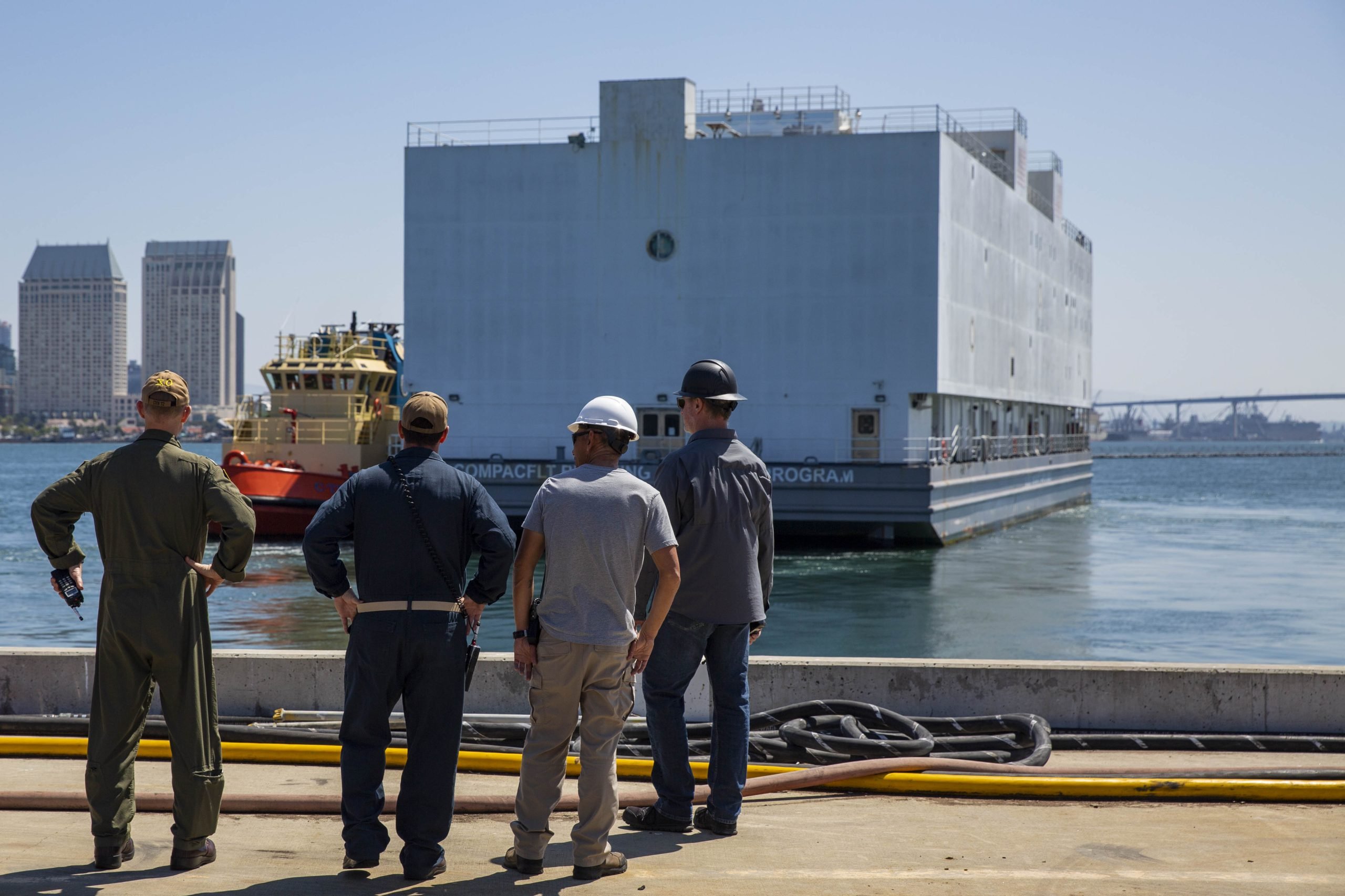In this captivating rectangular photograph of an outdoor scene, four construction workers stand on a concrete dock, their backs turned to the camera as they observe a massive ship departing the dock. The colossal square vessel, with fencing surrounding a structure on its top, towers approximately four or five stories high and is securely perched on a barge. To the left side of the ship, a vibrant red tugboat is visible, seemingly assisting the barge. On the far left, beyond the water's edge, a couple of buildings stand tall against the clear blue sky, suggesting a bay inlet setting. A large rope lays coiled in front of the workers, resting beside a low wall that borders the water. The entire scene is bathed in bright sunlight, enhancing the vivid colors and the tranquil atmosphere of this sunny day.